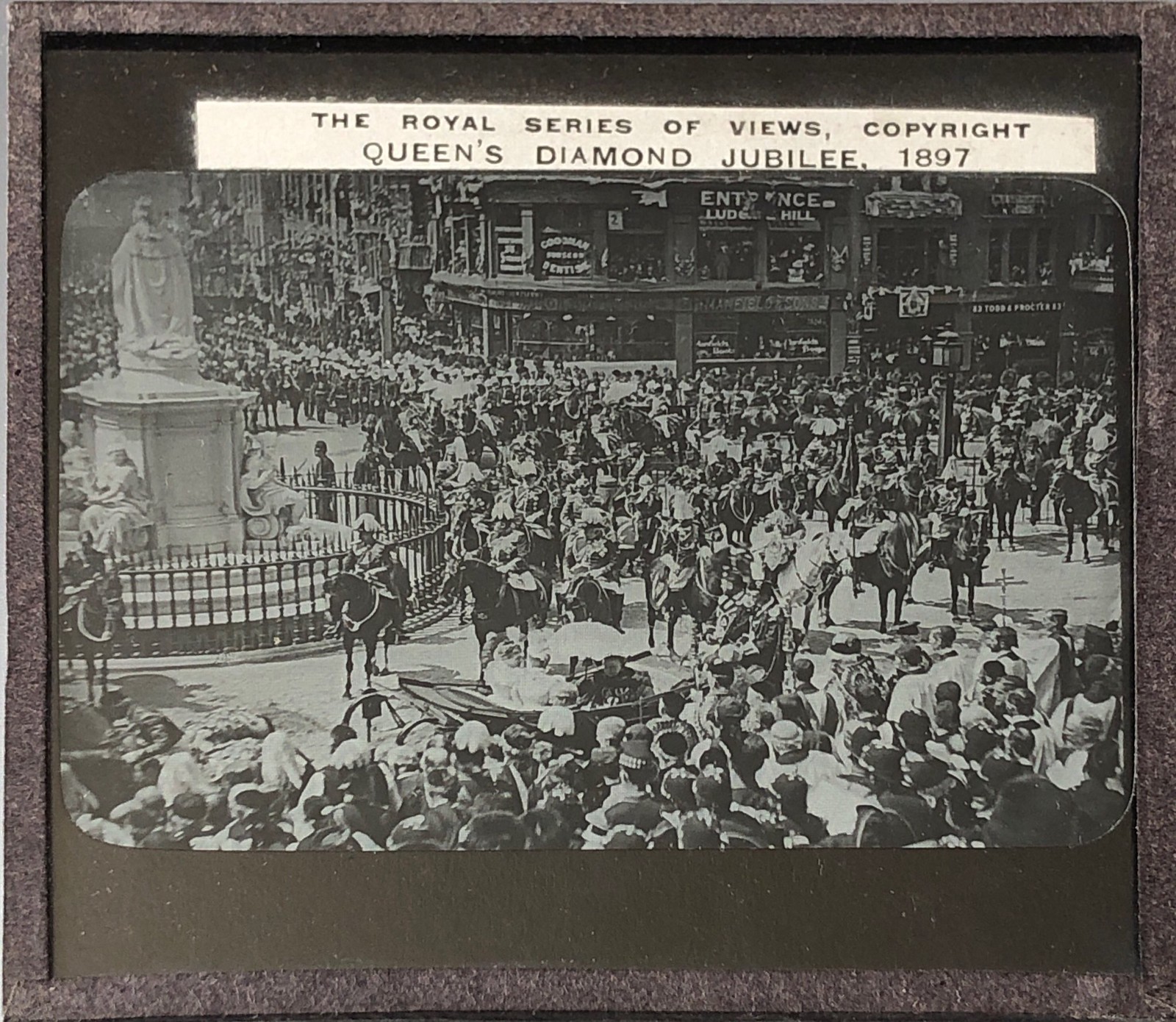This is an image of an old photograph, framed meticulously with a distinct border. The outermost edge features a thin light gray border, followed by a thinner black border on the top and left sides. Inside this frame, there is a thicker black matting at the bottom and top. Above the photograph, on white paper, is an inscription that reads: "The Royal Series of Views - Copyright Queen's Diamond Jubilee 1897."

The photograph itself captures a bustling town square, alive with the celebrations of the Queen's Diamond Jubilee. In the center of the image, there is a large statue mounted on a white base, approximately ten feet tall, surrounded by a round wrought iron fence. The statue, located on the left side, dominates the scene.

In front of the statue, several men on horses are aligned side by side, extending from the left to the right of the image. Behind them, a dense crowd lines the streets, filling both the foreground and background. Numerous storefronts with visible signs, a building marked with the word "Entrance," and a streetlight on the right, frame the festive atmosphere.

The photograph depicts the converging streets lined with an array of buildings, capturing the liveliness and grandeur of the occasion, though the Queen's caravan is not distinctly visible and may be obscured behind the horses in the center. The scene vividly epitomizes the jubilant spirit of the period celebration.